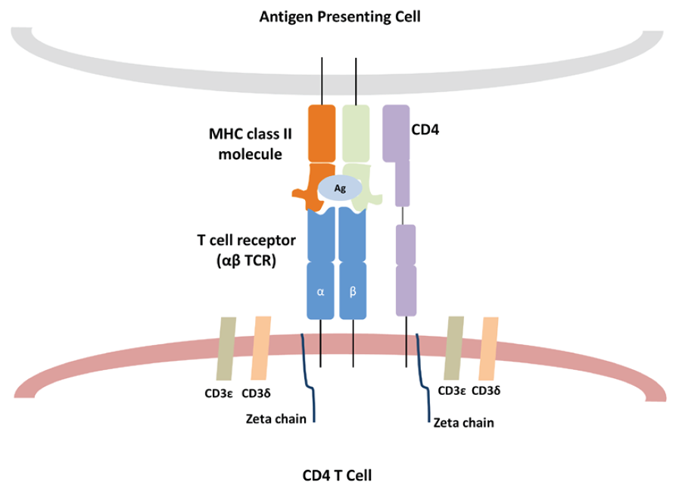This detailed medical schematic illustrates a cellular interaction involving an antigen-presenting cell and a CD4 T cell. At the very top of the image, in bold black letters, it reads "Antigen Presenting Cell." Just below this title, a light gray curved line arcs from the left corner to the right corner. Within this arc, there are two tubes: a brown tube labeled "MHC Class 2 Molecule" to the left and a light green tube similarly labeled.

Beneath the arc, three vertical, candle-shaped objects are visible. The leftmost vertical line has an orange top and is labeled "MHC Class 2 Molecule," with its bottom half colored light blue and marked as "T Cell Receptor" to the left. Adjacent to the orange top, "T Cell Receptor" is prominently mentioned. To the right, a segmented purple line is situated, labeled "CD4" at the top segment. Encompassed within the schematic, a gray line labeled "CD3," a flesh-colored line labeled "CD36," and two small blue thread-like lines known as "Zeta Chains" connect the sections. These elements are symmetrically repeated on both the left and right sides of the schematic.

The entire diagram shows a detailed interaction between the cell components, and at the bottom in black lettering, it specifies "CD4 T Cell." The visual emphasis includes crucial components like the antigen-presenting cell, various molecules such as MHC Class 2, CD3, CD4, CD36, and Zeta Chains, and their interconnected positions, providing a comprehensive overview of the cellular presentation system.